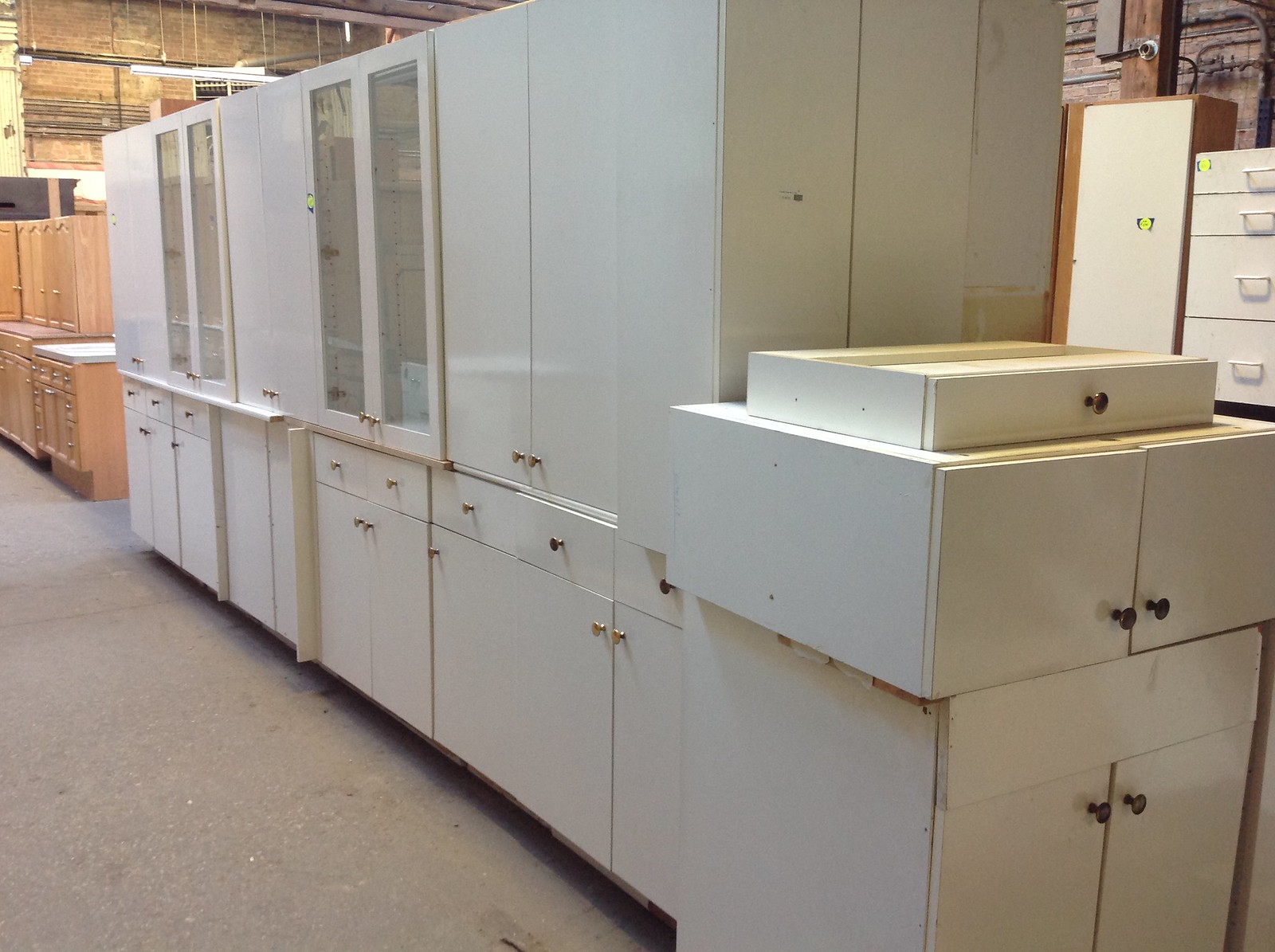This photograph captures the interior of a furniture showroom with a white cement floor arranged diagonally from the bottom right to the top left. Dominating the foreground are rows of white wooden hutch and dresser-type cabinets. Each white cabinet features simple, dark round knobs and some display glass panels running vertically in the center, with cabinet doors and drawers beneath. Toward the top left of the image, the color transitions to cabinets in a maple shade of wood, retaining a similar style but appearing less modern. Distinctly, there are two white cabinets with glass doors in the middle section. In the background, stacked high against the wall, are thick plywood sheets, reminiscent of a warehouse storage setup, adding a raw, industrial touch to the showroom ambiance.